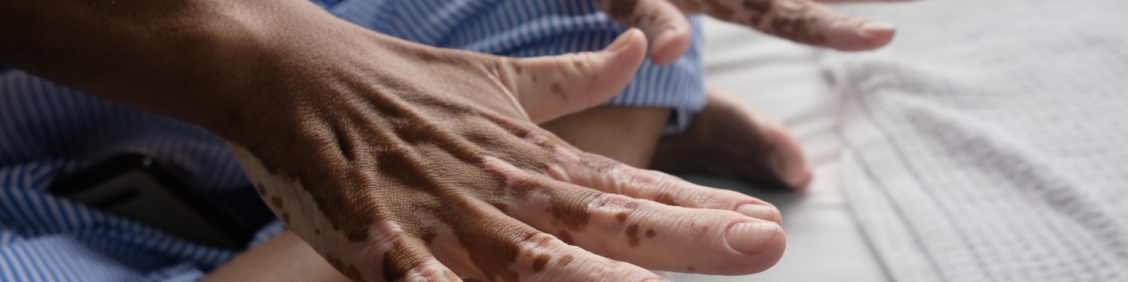This photograph captures a detailed and intimate look at a person's hands, emphasizing the unique skin pigmentation and setting. The right hand is prominently centered and in sharp focus, exhibiting a striking contrast of dark and light patches, possibly indicative of a skin condition or burn. The left hand appears in the background, slightly out of focus. The individual is dressed in blue and white pinstriped pajamas, suggesting they are seated, possibly with legs crossed, on a bed or sofa covered by a white blanket. The composition includes elements like the blue material and potential presence of a child's leg, adding to the complexity of the scene. Despite the photo's small dimensions of approximately 1.5 by 7 inches and an unusual crop, it vividly captures the central theme of the varied skin tones across the person's hands, posed straight out and seemingly under inspection. The image lacks identifying information about the subject or the photographer, focusing instead on the intricate details and textures presented.